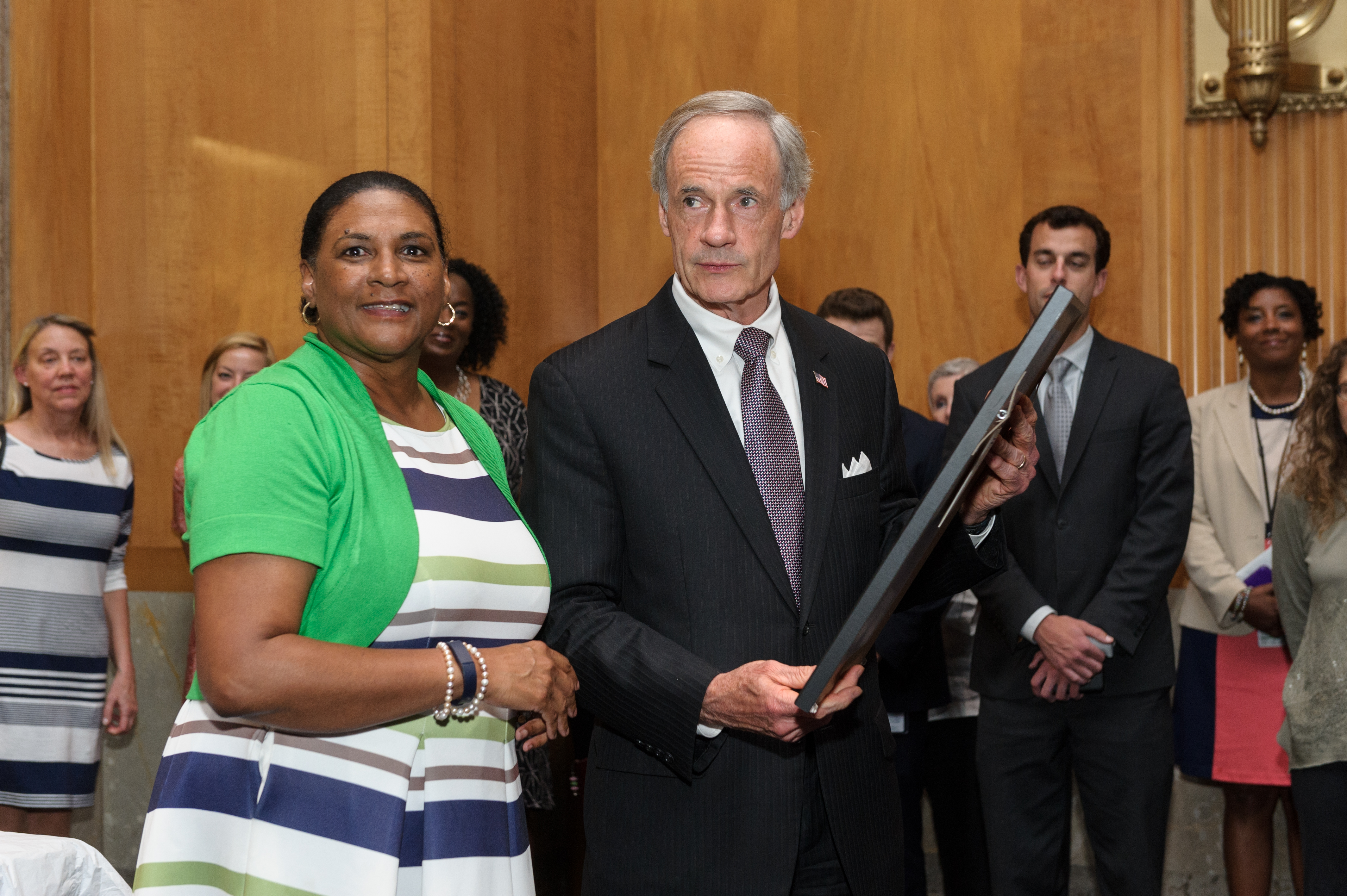The image depicts an indoor scene centered around a distinguished older white man and a black woman in the foreground, with several other individuals standing in the background. The man, who has short gray hair and looks like a familiar figure, possibly a senator, occupies the central position. He is attired in a dark-colored jacket adorned with an American flag pin, a white button-down shirt, and a purple tie. He holds a black picture frame, although the image inside isn't visible. The woman beside him is smiling, her black hair neatly tied back, and she wears hoop earrings. Her outfit consists of a blue, white, and green striped dress paired with a little green jacket. Both the man and the woman are positioned against a backdrop of light brown wooden paneling. The room is filled with a group of six to seven other people standing behind them, all contributing to the ambiance of the scene.